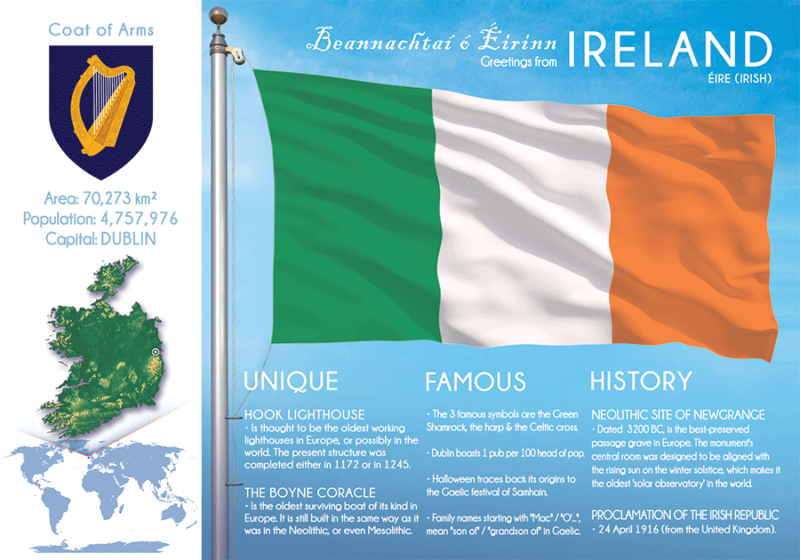The image is a detailed page about Ireland, divided into two main sections. On the left side, there's the coat of arms prominently displayed at the top, featuring a golden harp on a unique dark blue badge-like shield. Below the coat of arms, blue text details the area of Ireland as 70,273 square kilometers, a population of 4,757,976, and the capital city, Dublin. Further down, a green and yellow depiction of Ireland is shown, along with a location map illustrating Ireland's position in the world.

On the right side of the image, the Irish flag commands attention against a vibrant blue background, with "Ireland" written in large white text above it. The flag, attached to a metal pole on the left, appears to be fluttering in the wind, emphasizing its three stripes: green on the left, white in the middle, and orange on the right. Beneath these stripes are three sections labeled "Unique," "Famous," and "History" in white text, each accompanied by detailed descriptions. The "Unique" section highlights Hook Lighthouse and the bone coracle, while the "Famous" section lists Ireland's symbolic Green Shamrock, Harp, Celtic Cross, pubs, Halloween, and family names. Under "History," key historical notes include the Neolithic site of Newgrange and the Proclamation of the Irish Republic, with corresponding details. In addition, the top right corner also proudly displays the words "Beannachtaí ó Éirinn," meaning "Greetings from Ireland," in Irish.